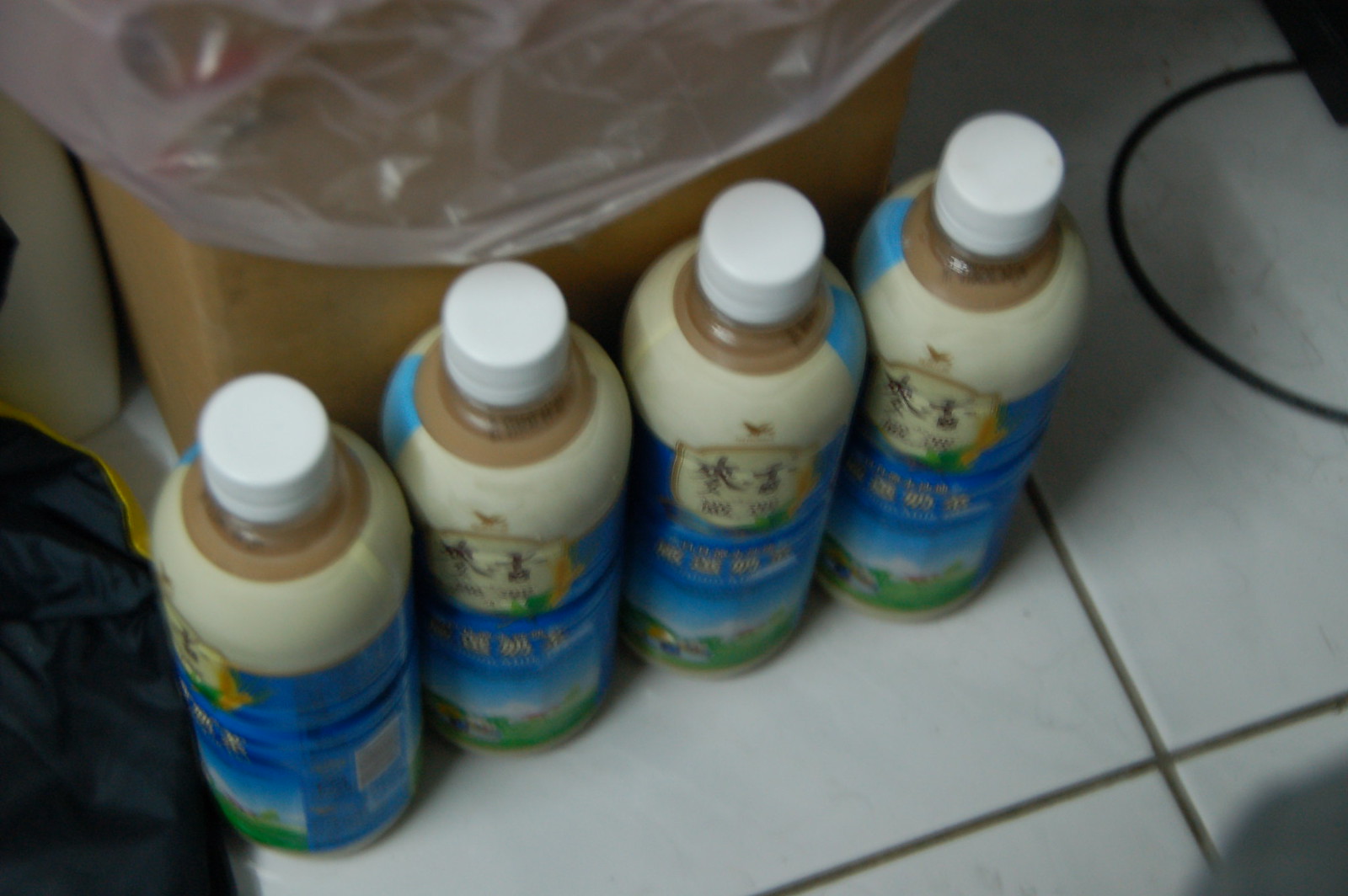The photograph, likely an older snapshot, shows four identical, unopened bottles with white tops that contain a brown liquid, possibly resembling chocolate milk. The bottles are adorned with Asian writing and small logos that are difficult to decipher due to the poor image quality. The bottle labels feature a cream color at the top transitioning to blue, with some green elements possibly depicting grass and a blue sky. The bottles are lined up on a grayish-white square tile surface with dark brown grout, suggesting it could be either a kitchen or bathroom countertop. Behind the bottles, there is a cardboard box with bubble wrap, indicating recent shipment. Also visible is a black cord and a brown trash can with a clear bag inside, adding context to the setting.